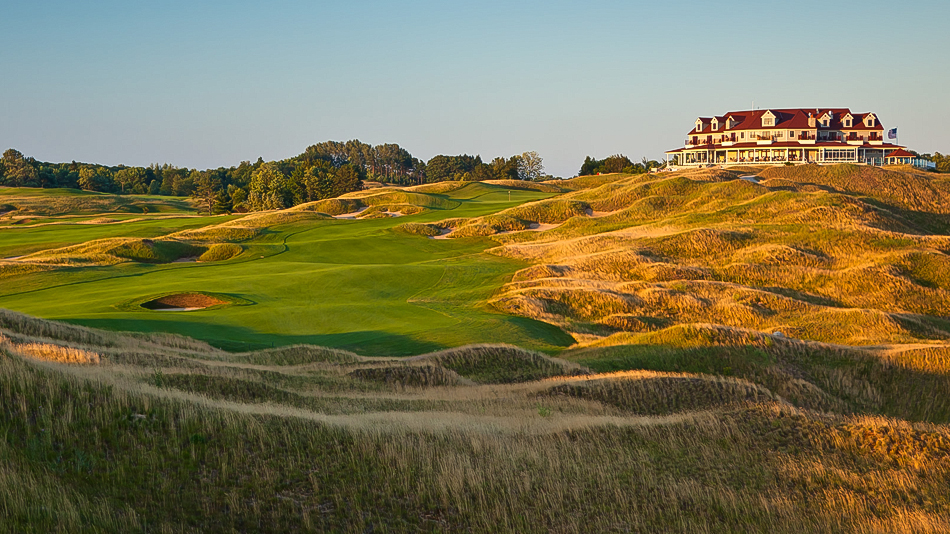The image showcases a picturesque golf course with a long fairway stretching across the scene, accentuated by rolling hills of rough terrain on the right. In the foreground, the grass transitions from long and green to a grayish-beige hue. Further back, on the left, a small sand trap lies adjacent to the dark green course where a flag can be spotted in the distance. Woods frame the left side of the background, enhancing the natural beauty of the setting. Dominating the upper right of the image, perched atop a hill, is a grand building resembling a luxurious resort or country hotel. This impressive structure features red roofs and cream-colored or white walls, spanning three stories with a veranda encircling the ground floor and multiple rooms, each with flower boxes under the windows. The second floor boasts additional flower boxes and windows, while the attic displays seven windows facing forward. The sky above is overcast with white clouds, suggesting a calm, daylight atmosphere.